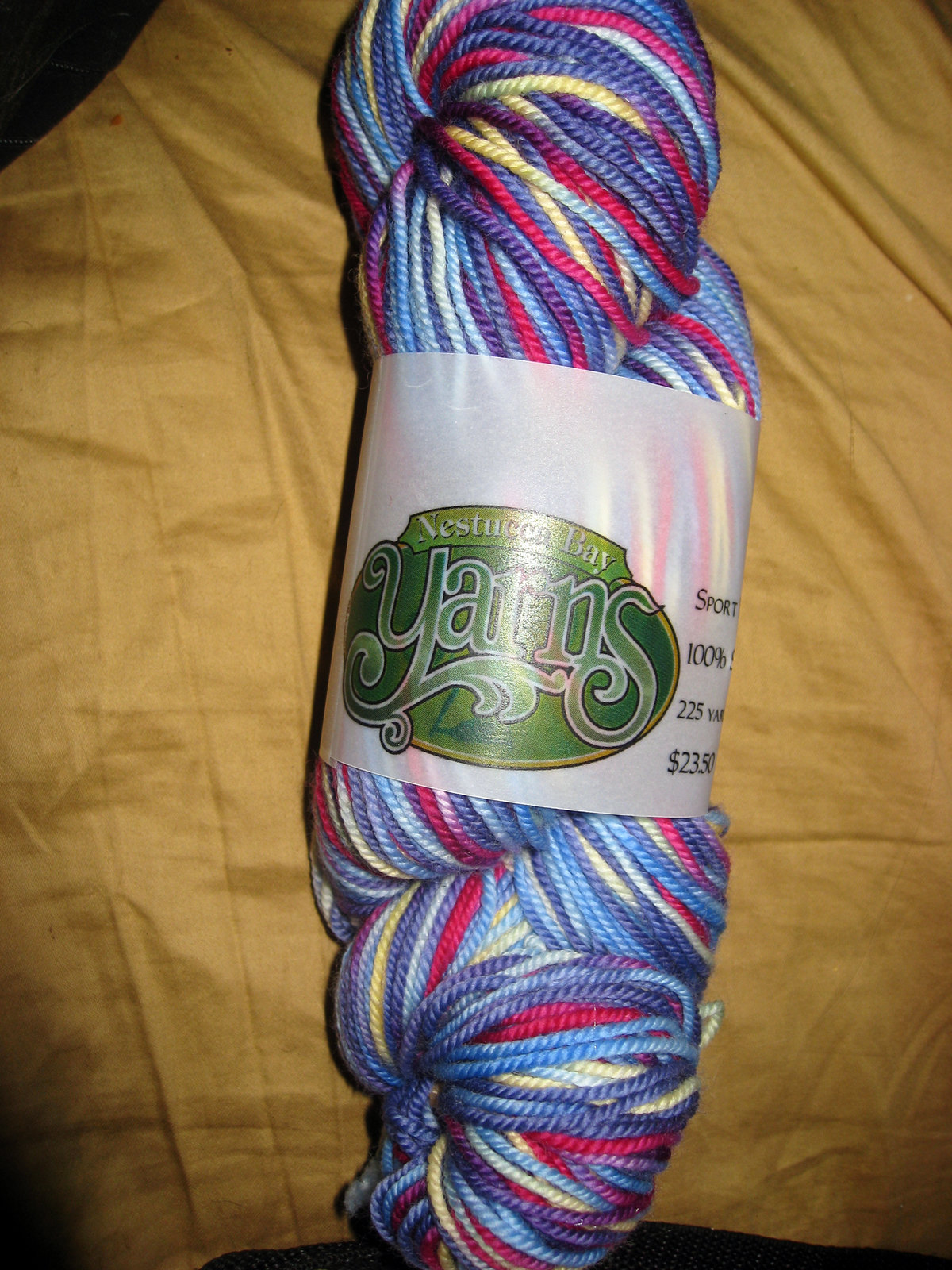This photograph features an unused roll of yarn, neatly wrapped in a clear plastic sleeve. The sleeve bears an oval-shaped green label adorned with the word "YARNS" prominently displayed across its surface. Above this, the label also includes the brand name "NEST", followed by additional text that appears to say "Cat Bay." The yarn itself is a vibrant, multicolored assortment, predominantly showcasing various shades of blue, with interspersed streaks of red, white, and yellow. The colorful roll of yarn is resting atop a cozy tan blanket, offering a warm and inviting setting.